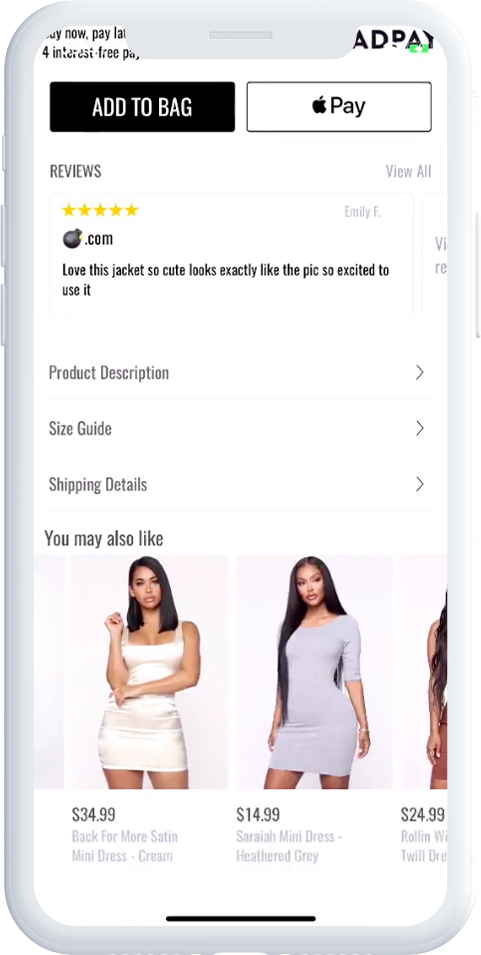The screenshot displays a mobile shopping site interface, showcasing options for purchasing a product. The user can make the purchase in four installments, with the option to use Apple Pay. Prominent on the screen is the "Add to Bag" button, accompanied by a five-star rating for a jacket. Below this, sections for "Product Description," "Size Guide," "Shipping Details," and "You May Also Like" are visible. The image also features two models: the first is wearing a cream-colored, form-fitting mini dress with a square neck and thin straps; the second model is dressed in a heather gray mini dress with three-quarter sleeves and a rounded neck. Although the user appears to be interested in a jacket, no jacket is visible in the screenshot.